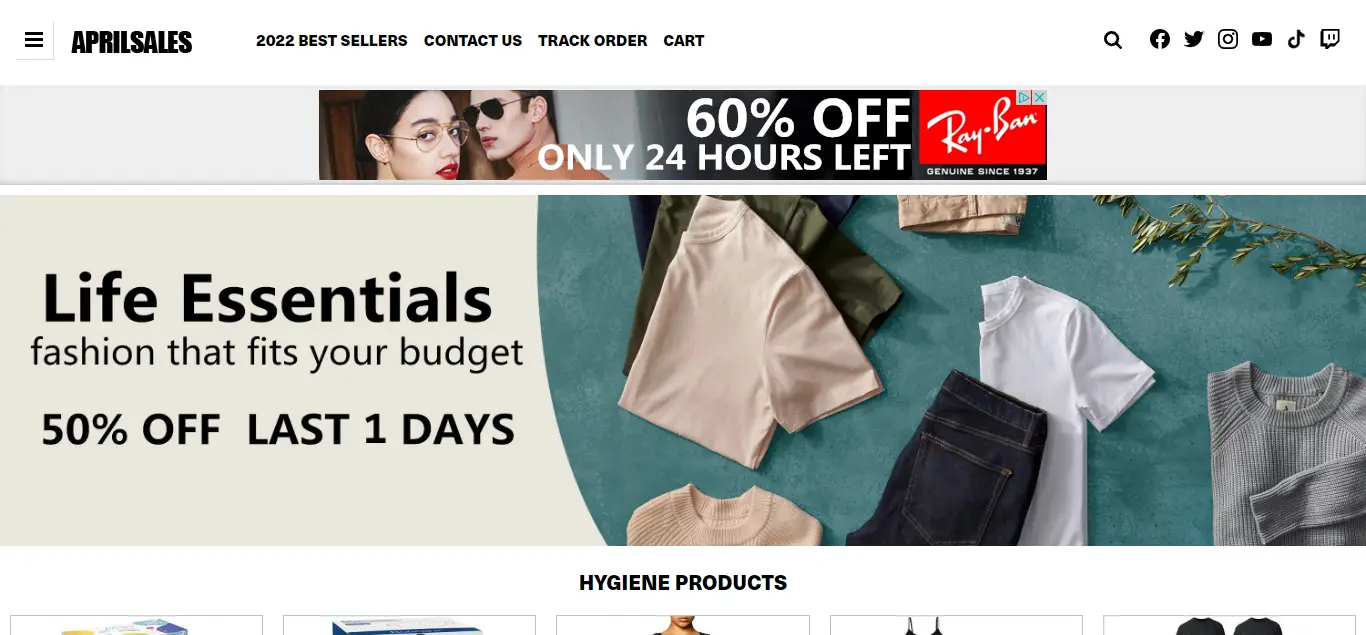This image, sourced from a website advertising April sales, features several prominent elements. In the upper right-hand corner, there are clickable options such as "2022 Bestsellers," "Contact Us," "Track Order," and "Cart." Adjacent to these, social media icons provide quick access to various platforms.

At the top center of the image, a bold red rectangle announces "60% OFF - Only 24 Hours Left," alongside the "Ray-Ban" brand name, distinctively formatted as "R-A-Y-B-A-N."

Moving to the middle section, a large text reads, "Life Essentials - Fashion That Fits Your Budget," followed by "50% Off - Last 1 Days." This section showcases a collection of clothing items, including a beige shirt, a green shirt, a beige sweater, and a pair of dark blue jeans laid next to a neatly folded white t-shirt. There is also a grayish, stonewashed sweater displayed.

Towards the bottom of the image, the caption "Hygiene Products" is present, with five boxes partially visible, indicating that the rest of the products are cut off in the image.